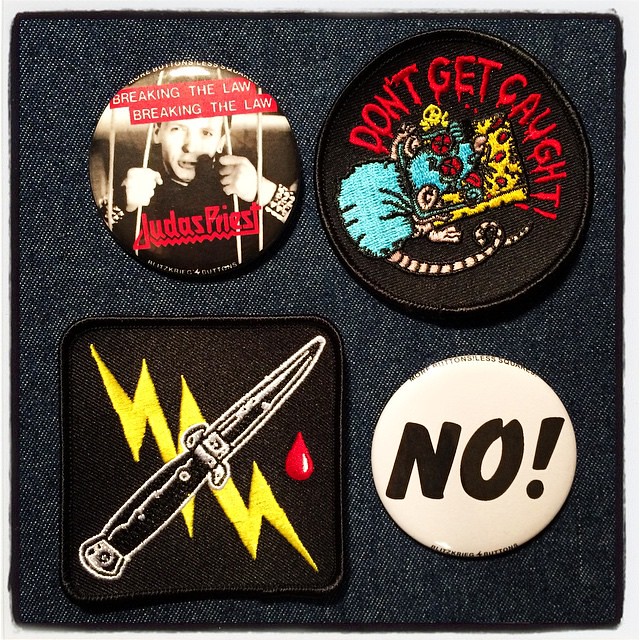This image depicts a dark, coarse square of denim fabric adorned with two patches and two pins. The denim appears dark blue or black, speckled with white. Starting at the top left corner, there is a circular pin illustrating a Caucasian man seemingly breaking out of jail; he is bending red bars with his hands adorned in studded wrist bracelets. The phrase "Breaking the Law, Breaking the Law" is written in white on red banners, and "Judas Priest" is inscribed in red below the man’s hands. To the top right, a round, black patch features the phrase "Don’t Get Caught" in red letters and depicts a blue rat with a bald tail, caught in a bright yellow mousetrap, its eyes disturbingly red and bulging. Moving to the bottom left, a black square patch presents an image of a lightning bolt and a detailed black knife highlighted in white, suspended in mid-air, with a red droplet poised near the knife's tip. On the bottom right, a white circular pin displays the emphatic word "No!" in big, bold, black letters against its stark background.